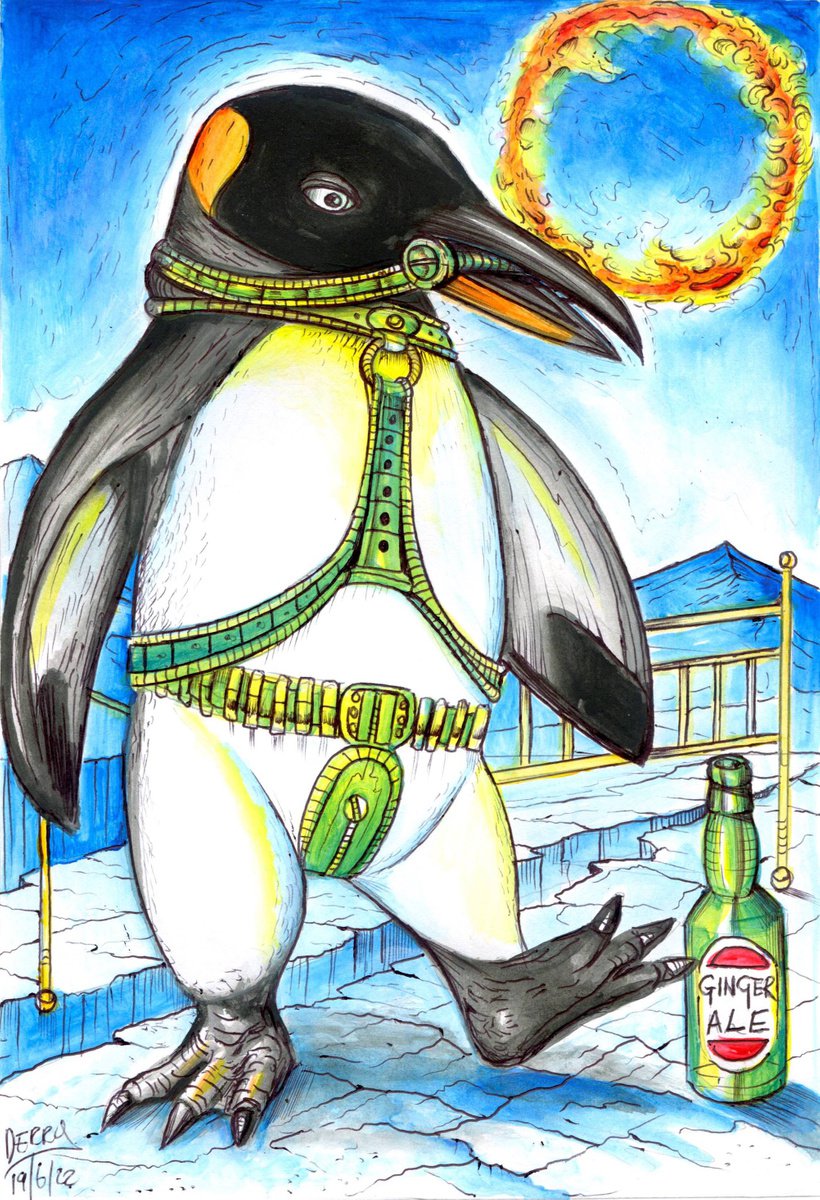The hand-drawn cartoon image depicts a tall, formidable penguin set against a predominantly blue, icy landscape that evokes a cold climate reminiscent of Antarctica. The background is filled with icy mounds and a bright blue sky, punctuated by a striking, flaming orange ring to the right side of the image. This ring appears to be composed of fire, with vibrant hues of orange and yellow. 

In the foreground, the penguin stands as the central figure, appearing almost like a superhero. It has black wings with white undersides and yellow stripes, a white belly with additional yellow stripes along the sides, black claws on its feet, and a black head marked by an orange spot on the back. The penguin's beak is black on top and orange on the bottom, holding what seems to be a piece of metal wire or tubing, which extends into a green harness-like apparatus. This harness fits snugly around its neck and torso, resembling a horse's reins or a complex piece of tactical gear, complete with a belt and a zipper around its lower half. The penguin’s right leg is lifted, suggesting movement, as it stands on a cracked icy surface.

Behind the penguin, a golden or yellow gated structure, akin to a metallic bedpost, adds a mysterious element to the scene. Additionally, a green bottle labeled "ginger ale" lies near the penguin's raised right leg, adding a touch of everyday whimsy to this fantastical tableau. The combination of these vivid details creates a dramatic and intriguing scene that blends elements of the surreal and the heroic.